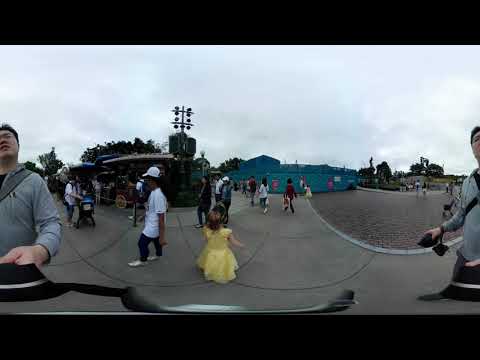In this detailed image, a 360-degree photograph captures a bustling urban plaza. The focal point is an individual, likely Asian, wielding a selfie stick with a GoPro that creates a mirrored effect, showing them on both edges of the image. The person is clad in a bluish sweatshirt, extending their left arm, which appears again on the opposite side. The visual is slightly morphed at the bottom due to the 360-degree stitching.

The setting is a busy street scene featuring a mix of smooth concrete and cobblestones or brick paving. Various people populate the scene, ranging from older adults to young children. Prominently, a little girl in a yellow dress walks away from the camera in the foreground. Many passersby are carrying shopping bags, suggesting a shopping district or market area.

The left side of the photo reveals what appears to be an open-air market or a series of booths, while the background showcases a long, single-story blue building or wall. Further in the distance, trees are visible, adding depth to the urban landscape. The sky above is heavily overcast, contributing to the overall atmosphere of the photograph.